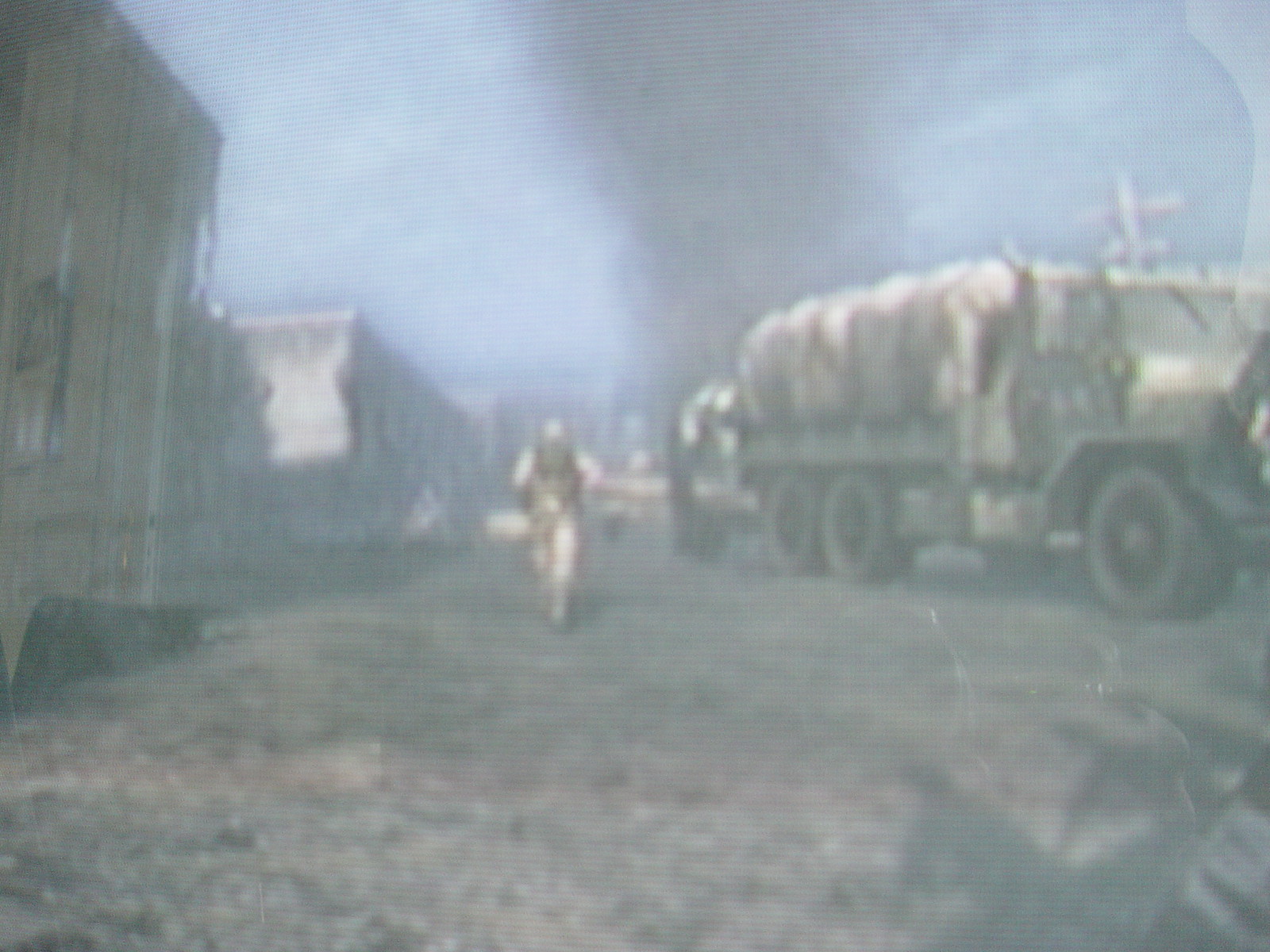In this blurry and grainy image, we are presented with a scene that resembles a war zone. On the right side of the photo, there is a large military vehicle, possibly a cargo or transport truck, characterized by its multiple tires and covered back area. This vehicle appears yellowish with hints of green. In the center of the image, a lone figure dressed in military attire, perhaps a yellowish-beige or camouflage uniform, is visible. The soldier, who seems to be carrying a backpack, is walking away from the camera. The scene is filled with a haze, dominated by a substantial plume of gray smoke rising into the otherwise blue sky, potentially indicating the aftermath of a recent explosion. Additionally, a telephone pole is faintly discernible on the right-hand side, adding to the chaotic yet structured environment of the photograph.